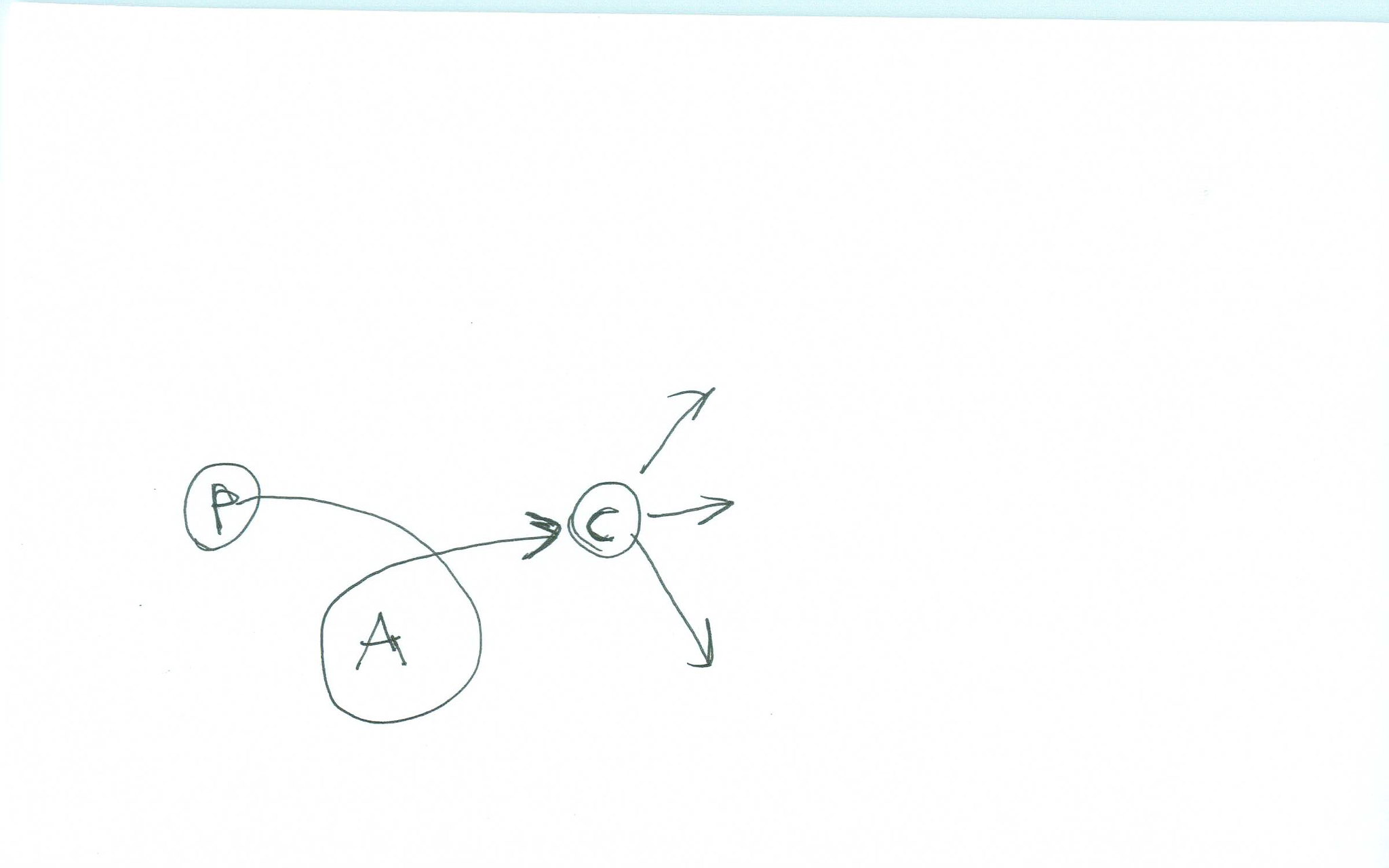The image presents a diagram set against a white background, illustrated with black ink. The diagram features three circles, each labeled differently: 

- Circle B is positioned on the left side. 
- Circle A is located at the bottom. 
- Circle C is on the right side.

There's a curved line connecting Circle B to Circle A. Another line extends from Circle A towards Circle C with an arrow pointing towards Circle C, indicating direction. Circle C further has three arrows emanating from it, pointing in three distinct directions: one pointing straight ahead, one pointing upwards, and one pointing downwards.

This figure appears to represent a geometric or possibly mathematical concept, with the detailed connections and directional arrows providing a clear relational structure among the circles A, B, and C.